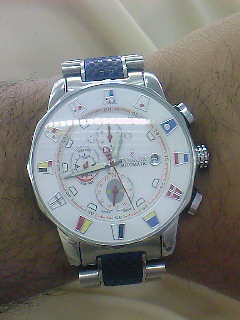This close-up photograph features an ornate wristwatch worn on the wrist of an individual with olive-toned skin, suggesting they might be Caucasian or Hispanic. The person, who possibly has dark hair and appears to be male, has positioned their hand over a white sheet, creating a soft, neutral background for the shot. The watch itself is intricately designed, boasting a white face adorned with flags of various countries, one of which could be Ukraine. The watch face is detailed with additional smaller dials, enhancing its elaborate appearance. The band of the watch is predominantly silver, accentuated by striking blue links that connect the metallic segments. Only a small portion of the wearer's wrist and hand are visible, ensuring the watch remains the focal point of this detailed and visually captivating image.